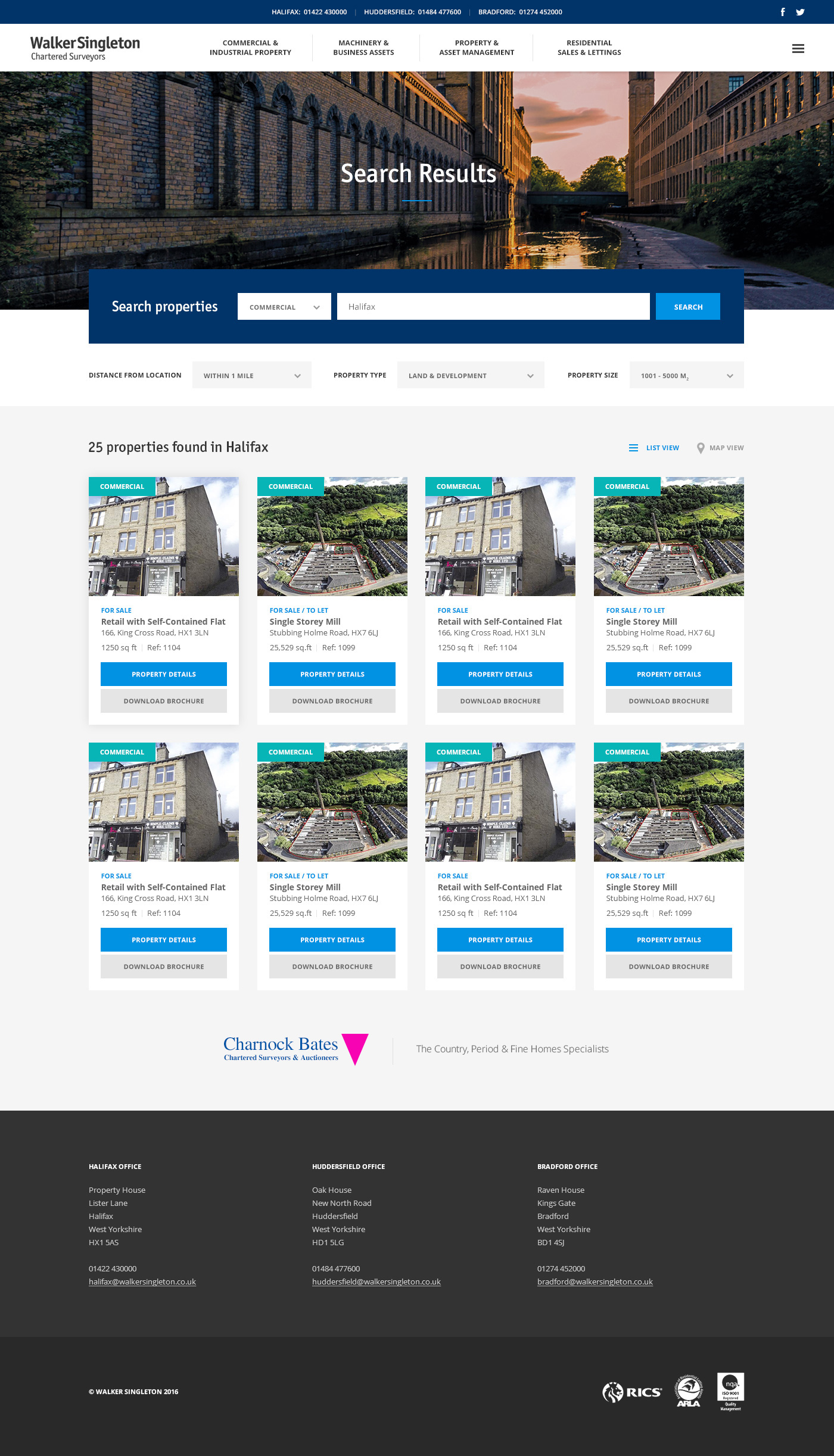In the image, the upper section features a blue background with concise text listing phone numbers for Halifax (0142234000) and Huddersfield (Bradford). Beneath this, the background shifts to white, where the left side hosts the logo and name "Walker Singleton Chartered Surveyors." This section also includes tabs for different services: "Commercial and Industrial Property," "Machinery and Business Assets," "Property and Asset Management," and "Residential Sales and Lettings."

Further down, the main content area is highlighted by the text "Search Results" atop a background image of a building adjacent to a lake. Below this, a blue search box prompts users to "Search Properties and Commercial Halifax," accompanied by a blue search button. Additional filtering tabs are provided, offering options like distance, location, property type, and property size.

The search results indicate "25 properties found in Halifax," with options to view them in either list or map format, though the list view is currently selected. Each property listing, designated for sale, includes two buttons: a blue "Property" button and a grey "Download Property" button. Notable listings include "Retail with Self-Contained Flat," "Single Storey Mill," and various flats either for sale or to let.

At the bottom left, the image features "Charnock Bates Chartered Surveyors and Auctioneers" alongside a pink downward-facing triangle. The footer, set against a black background, lists contact information for the Halifax and Bradford offices.